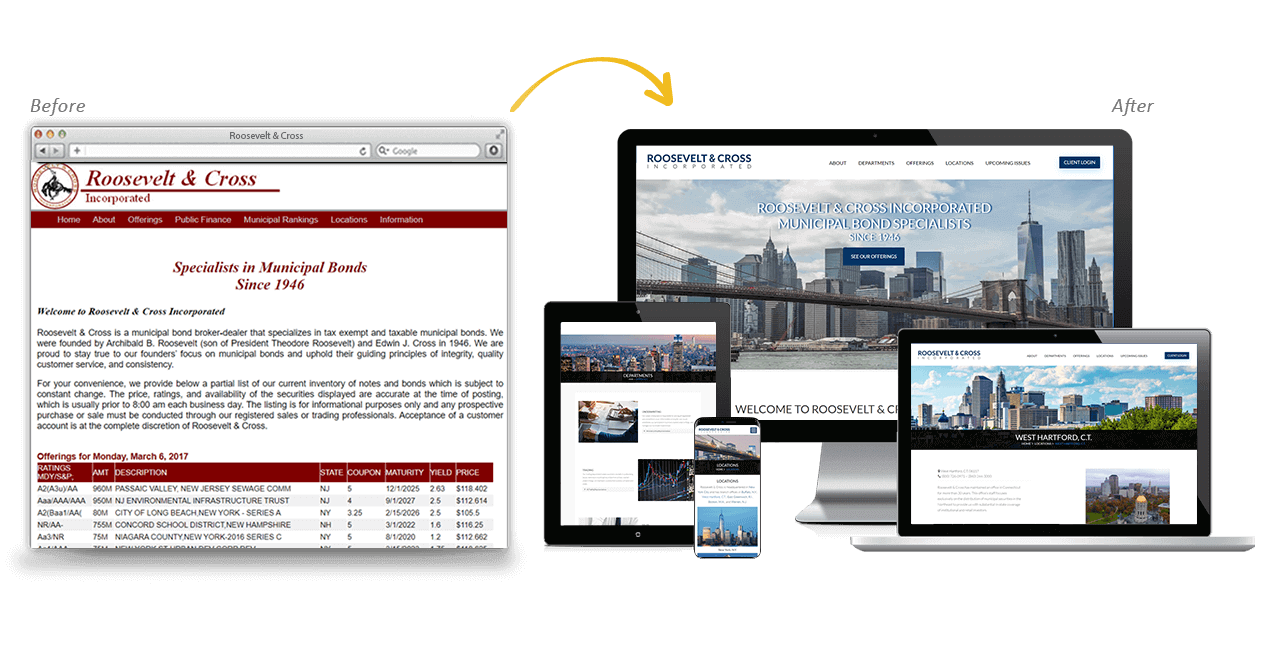The image is divided into two sections, each showcasing a different version of the Roosevelt and Cross website. The left section, labeled "before," displays an outdated, red-and-white themed website with black text on a Mac device. The design appears antiquated and less visually appealing. 

An arrow points from this old design to the new version presented on various devices, including a tablet, mobile phone, laptop, and an iMac. The right section, labeled "after," highlights a modern, white-and-blue themed website titled "Roosevelt and Cross Incorporated" in the upper-left corner. This updated design features several navigational tabs at the top, a prominent blue button on the upper right, and a background image depicting a city skyline with a river and bridge, giving it a fresh and professional look.